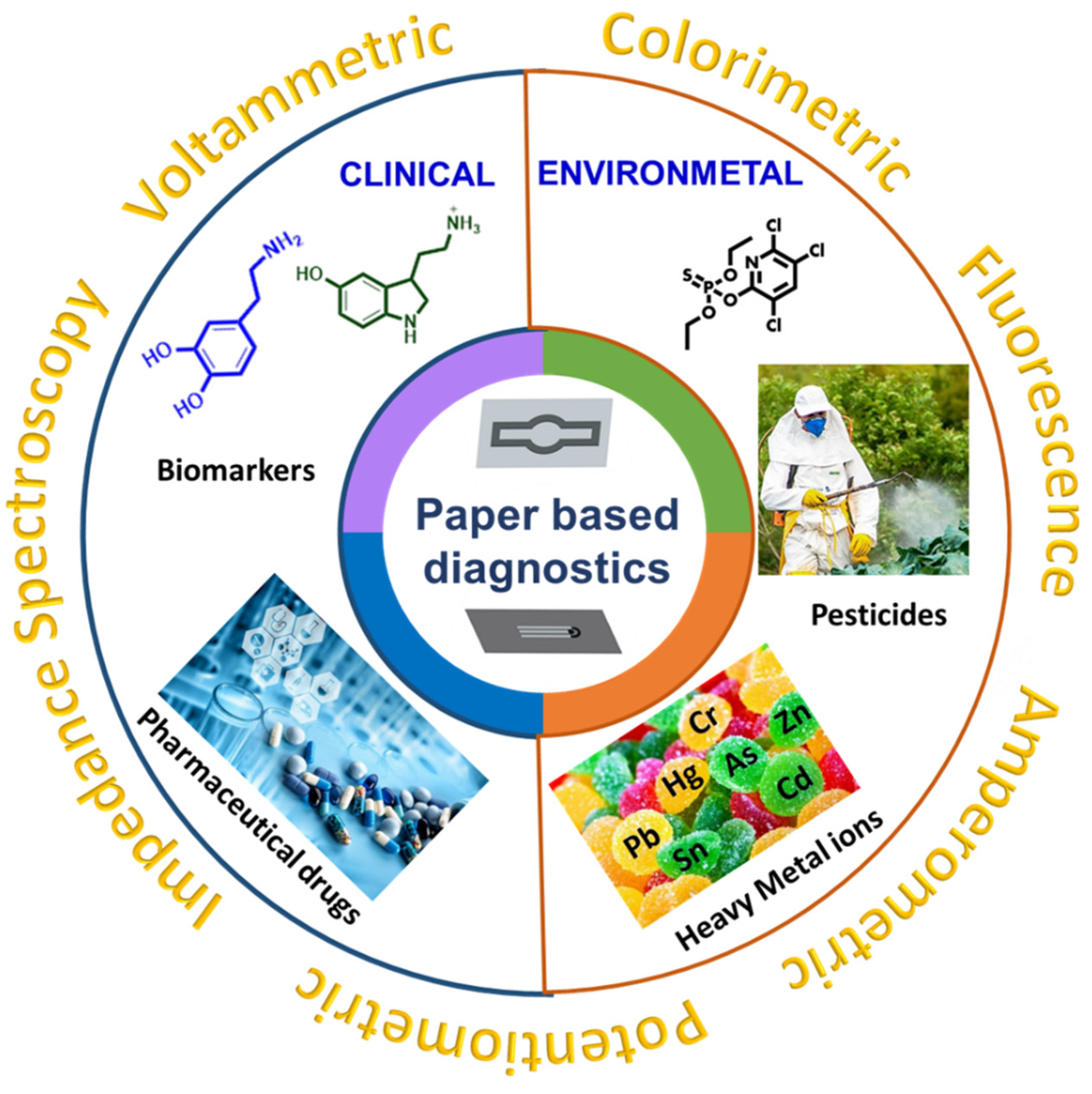The image is a detailed infographic designed in a circular format, divided into four distinct quadrants for clarity. Surrounding the outer perimeter of the circle are yellow-colored labels specifying different analytical techniques including voltammetric, colorimetric, fluorescence, amperometric, potentiometric, and impedance spectroscopy. 

Towards the center of the circle is another concentric circle divided into equal quadrants colored in pink, green, orange, and blue, with the central text reading "paper-based diagnostics." 

At the top inside the main circle, in blue text on the left side, it says "Clinical" and on the right side, it says "Environmental." 

On the left side, there are two chemical diagrams—one in green and another in blue—with the label "biomarkers" beneath them. Below this, there's a section labeled "pharmaceutical drugs," accompanied by an image of various pills on a blue table.

On the right side, a black chemical diagram is labeled "pesticides," illustrated with a photograph of a person spraying pesticides. Below this, there's another section labeled "heavy metal ions," represented with an image of jellybeans or gumdrops marked with chemical symbols such as Cr, As, and Cd.